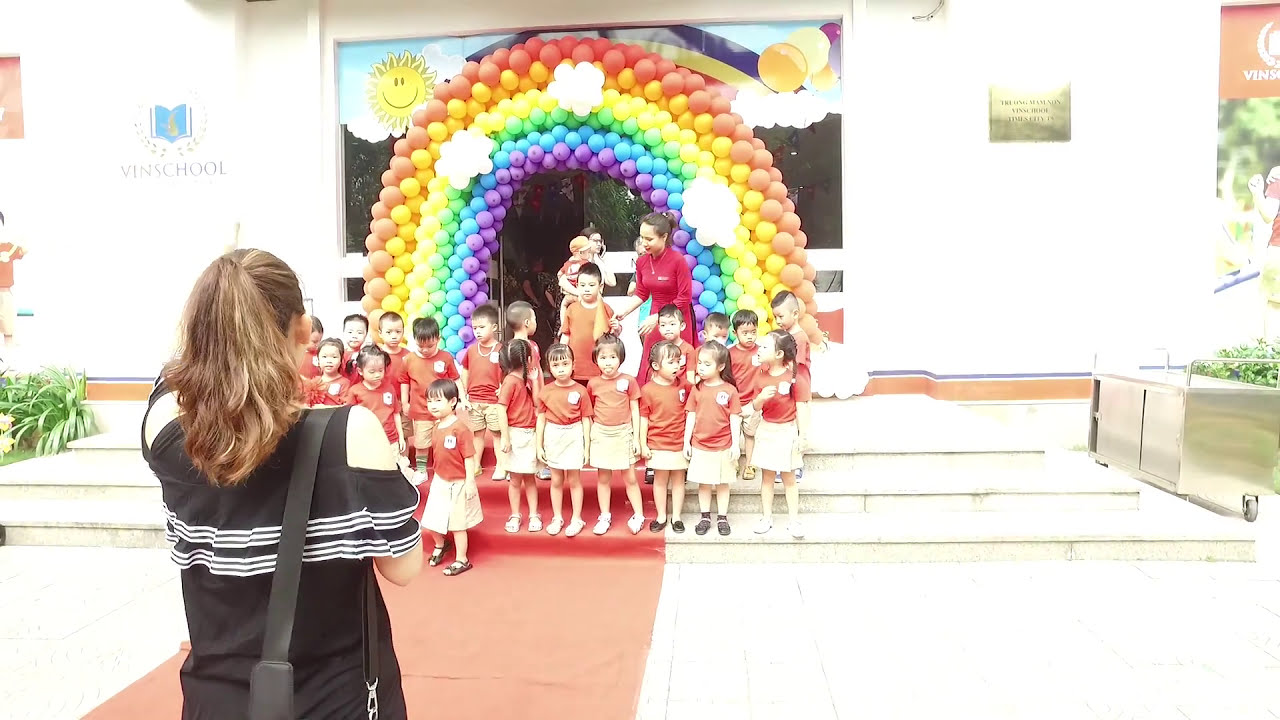The image depicts an outdoor scene on a bright day, highlighting a group of young children, likely preschool or kindergarten age, posing for a photograph. They are standing in front of a vibrant, ballooned rainbow arch, which forms an upside-down horseshoe shape featuring colors red, orange, yellow, green, blue, and purple. The children, both boys and girls, are dressed in uniform orange tops and beige skirts or shorts. Behind them, a taller woman, possibly their teacher, wears a red dress. Positioned with her back to the camera, another woman dressed in black appears to be taking the photo. The backdrop includes a white wall adorned with a cheery mural of a smiling sun in a blue sky, as well as a gold or bronze plaque with unreadable dark writing. In the upper left corner, the name of the school, "Venn School," is visible in darker gray writing on a blue book, suggesting a vibrant and educational environment.